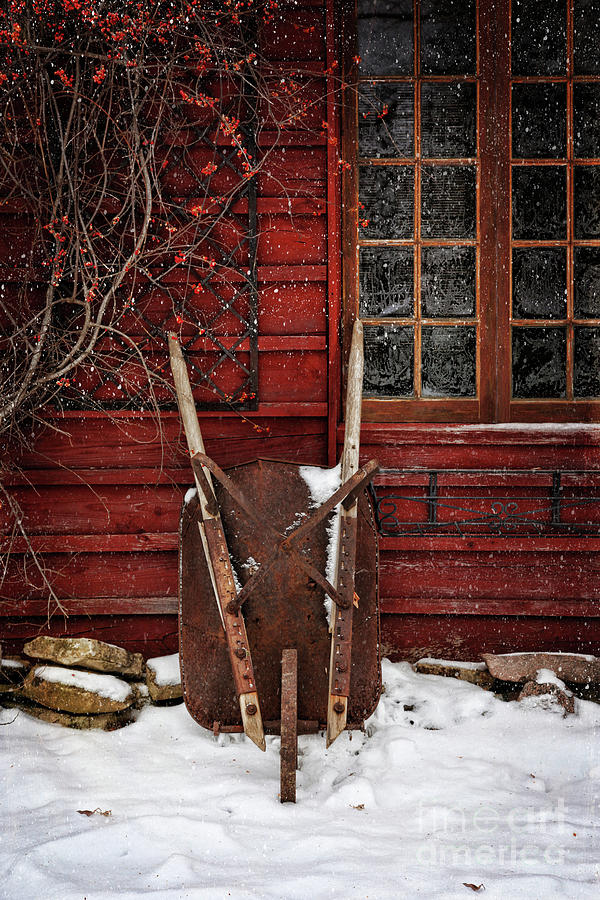In this elegant and classic winter scene, a rusted, brown wheelbarrow stands tilted up against the red exterior of what appears to be a cozy cabin or home, with its metal part visibly worn. The snow-covered landscape enhances the enchanting, Christmas-like atmosphere, with delicate holly berries adding a pop of reddish color amidst the predominant browns and whites. The black windows of the cabin, outlined by accumulating snow, add a charming touch to the rustic setting. Surrounding the wheelbarrow and the cabin, rocks peek through a blanket of snow, while a small bush or tree with budding flowers adds a hint of life to the otherwise serene tableau. There is no visible sky in the image, focusing on the intimate, close-up view of the wintery scene, and a nearly transparent "Fine Art America" watermark subtly rests at the bottom.